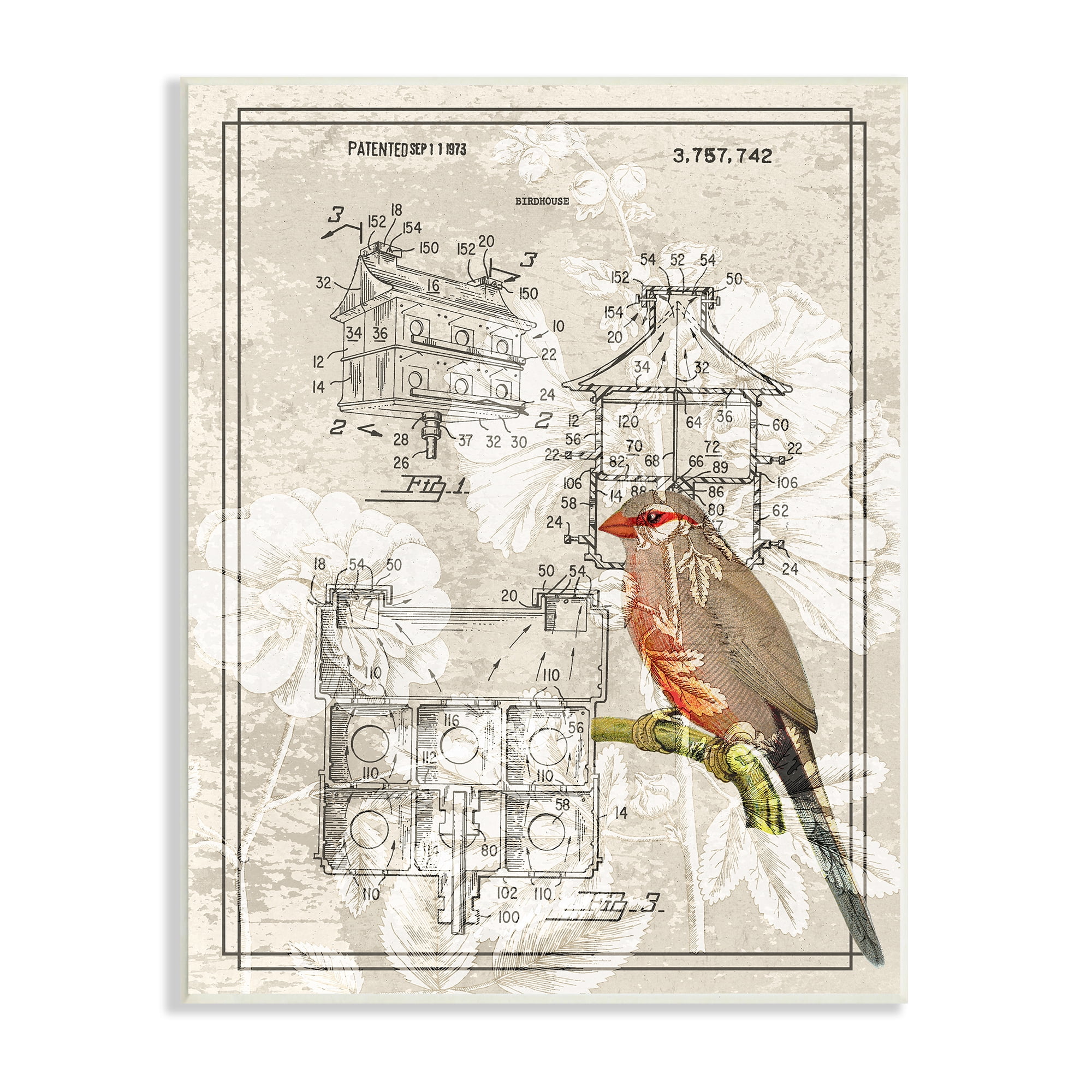This image appears to be a schematic for a patented birdhouse, with the patent dated September 11, 1973, and numbered 3,757,742. At the top of the page, it identifies the design as a "very small block type birdhouse." The page includes four images: three detailed schematics of the birdhouse from different angles, each labeled with numbers for clarity, and an illustration of a bird perched on a branch. The bird, which possesses predominantly brown feathers with some red and gray tones, is small and resembles a parakeet, although the exact species is not clear. The entire page has a decorative background featuring white flowers on a light brown or off-white base, lending a peaceful and picturesque quality to the technical drawings.